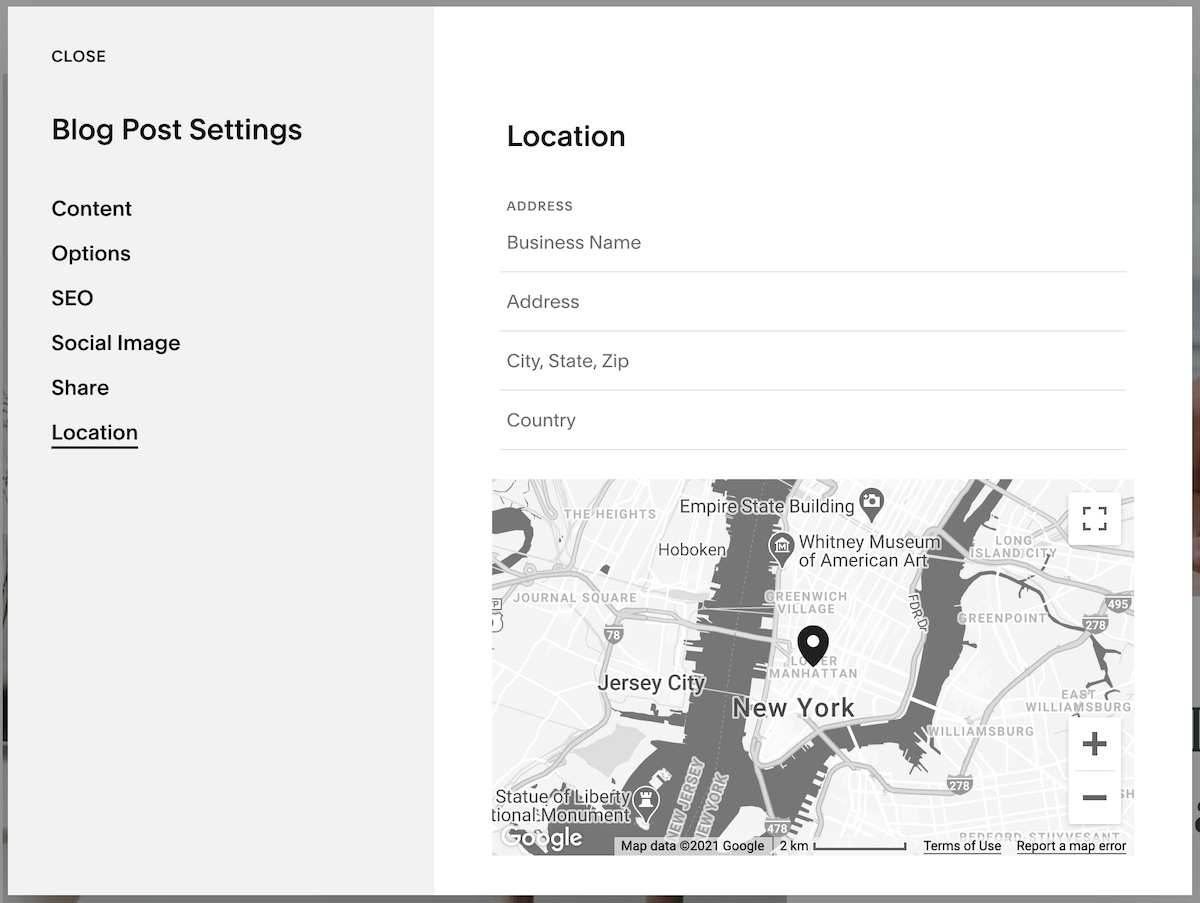The image is a detailed screenshot of the settings section of a website. At the top-left corner, a "Close" button is prominently displayed. Directly below this, a heading reads "Blog Post Settings," under which several options are listed: "Content," "Options," "SEO," "Social Image," "Share," and "Location."

On the right-hand side of the screenshot, another section is labeled "Location." Beneath this, fields for entering address details are displayed, headed by "Address." These fields, shown as empty text boxes, include inputs for "Business Name," "Address," "City," "State," "Zip," and "Country."

Lower in the image, a map is featured, zoomed into a section of New York City. Notable landmarks such as the Whitney Museum and the Empire State Building are visibly marked as locations on the map.